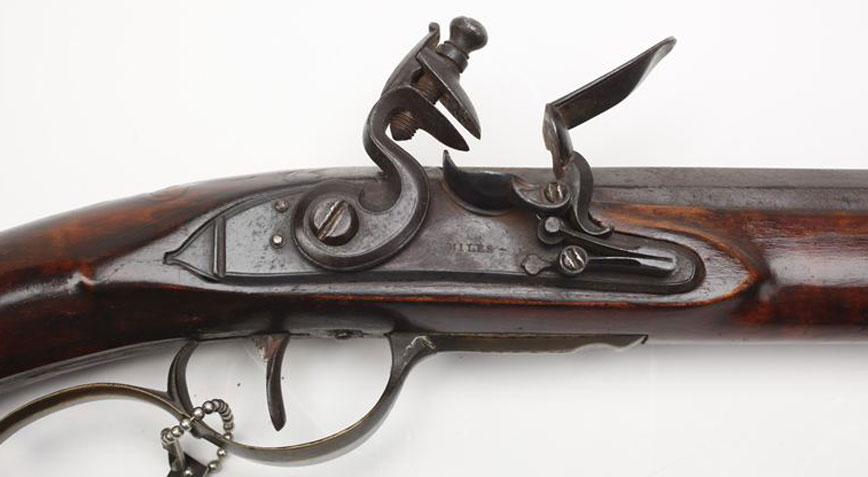This detailed close-up photo captures the central part of a flintlock rifle, prominently featuring the intricately designed metallic trigger and trigger guard. Part of the main body of the rifle is visible, showcasing dark brown wood that appears well-maintained and possibly stained, giving it a smooth, reflective finish. Small metallic details, including a chain near the trigger guard, add to the firearm’s ornate craftsmanship. The stamped name "MILES" is noticeable on the metal hardware, highlighting its historical value. The rifle points to the right against a light gray, possibly white, rectangular background, emphasizing the detailed workmanship and preservation of this likely British design.